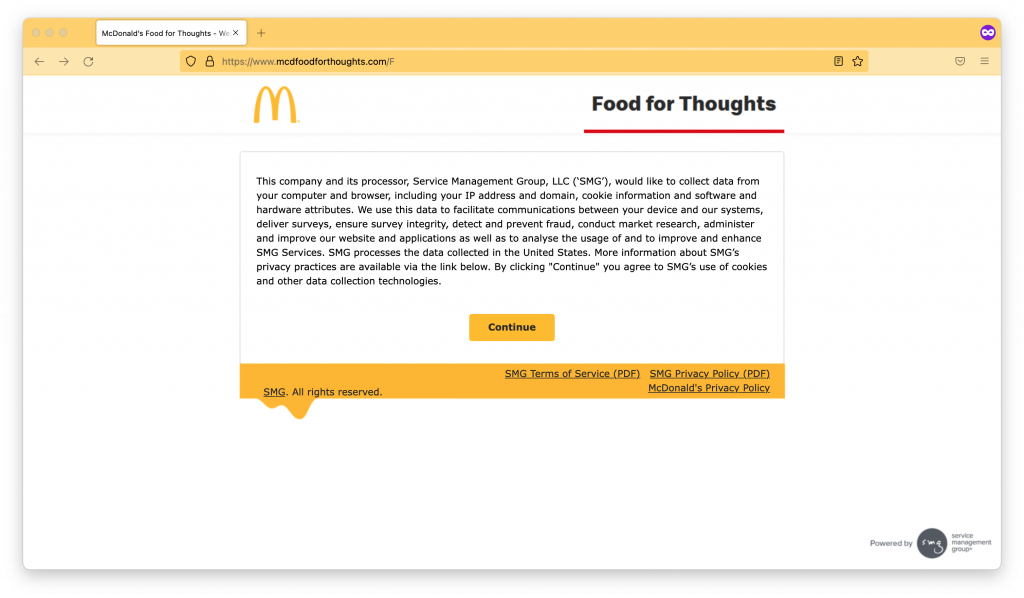This is a detailed description of a screenshot from a McDonald's webpage. The top of the page features a prominent orange border that extends across the top and down the far left side. In the far left, within the orange border, there is a text box displaying the phrase "McDonald's Food for Thoughts." Below this text box, the address bar is visible, showing the URL "www.mcfoodforthoughts.com."

The main body of the webpage has a white background. Centrally aligned towards the middle of the page is the iconic McDonald's logo, the golden arches represented by the letter "M." To the right of the logo, there is the phrase "Food for Thoughts" written above a red line. Beneath this phrase, a rectangular section with a white background and a slim gray border contains important information. The text within this rectangle states that the company, along with its processor, Service Management Group, LLC, seeks to collect data from the user's computer and browser. This data includes the IP address, domain, cookie information, and software and hardware attributes. The collected data is used to enhance communication between the user’s device and McDonald's systems, ensure the integrity of surveys, prevent fraud, conduct market research, and improve the website.

Under this information box, there is another rectangle with an orange background that contains the word "Continue" in bold text, prompting users to proceed. The bottom of this box has a thin orange border, which includes links to the "SMG Terms of Service" and "McDonald's Privacy Policy." In the bottom right corner, the page indicates that the site is "Powered by Service Management Group."